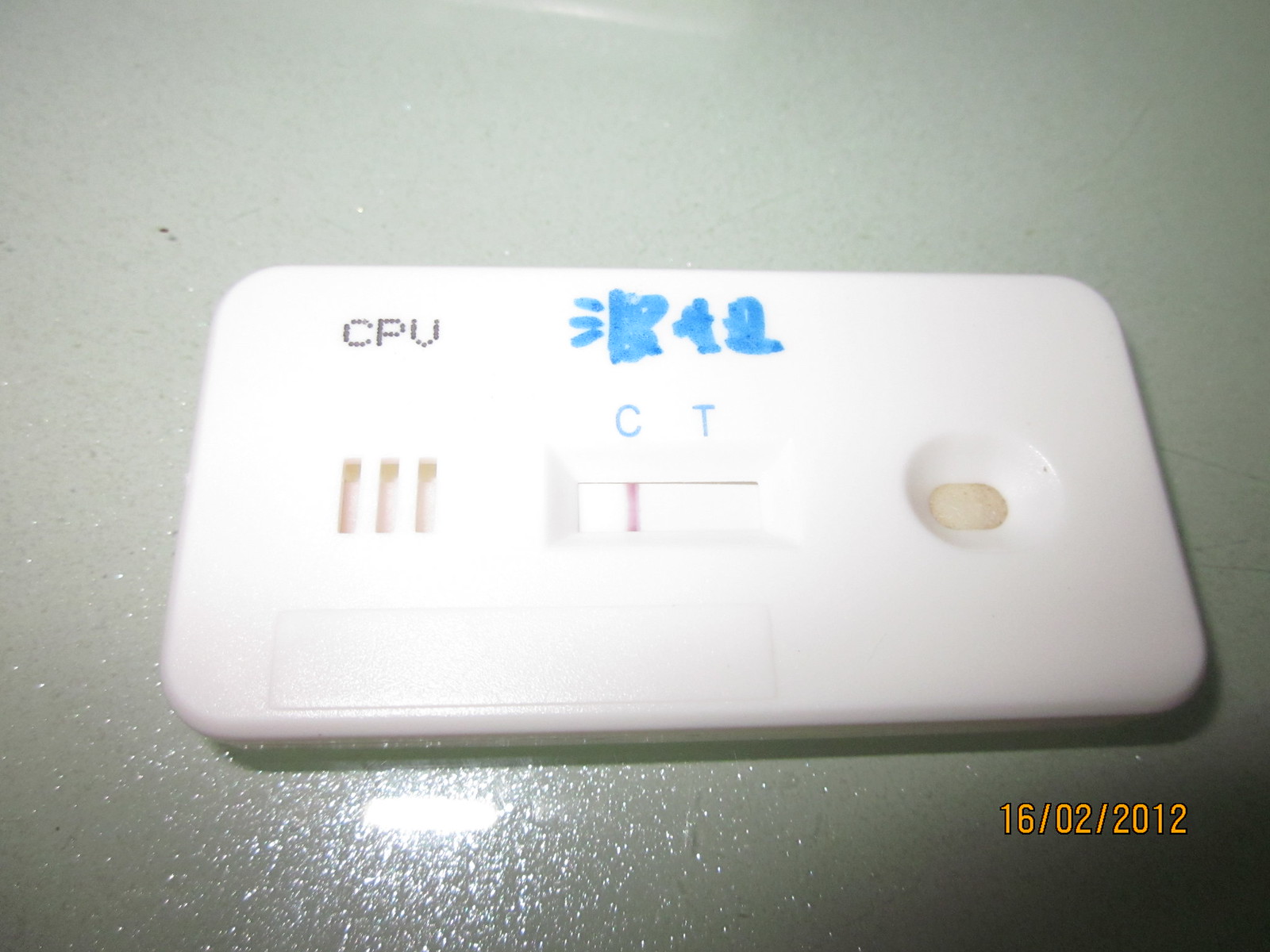This photograph features a compact, rectangular device with rounded edges. The device is predominantly white and fits comfortably within the palm of a hand, indicating its small size. At the top left corner, there is text that reads "CPU" in black, dotted lettering. Above this, slightly smudged blue text spells out "R42." Three horizontal lines are positioned to the left of the "R42" text, aligned with the left edge of the device. Directly below this, the text "CT" is inscribed, potentially indicating different test markers.

The central portion of the device contains a white, horizontal bar with a red line running through it, possibly serving as an indicator. This configuration suggests the device may be used for diagnostic purposes, such as testing for dental conditions, scientific analyses, or the detection of diseases. To the left of this white bar, there are three additional horizontal lines. On the right side of the device, a small button or light is present, which could serve as a functional component for operating the device or signaling test results. The overall design and markings imply this device is a sophisticated tool for some form of medical or scientific testing.